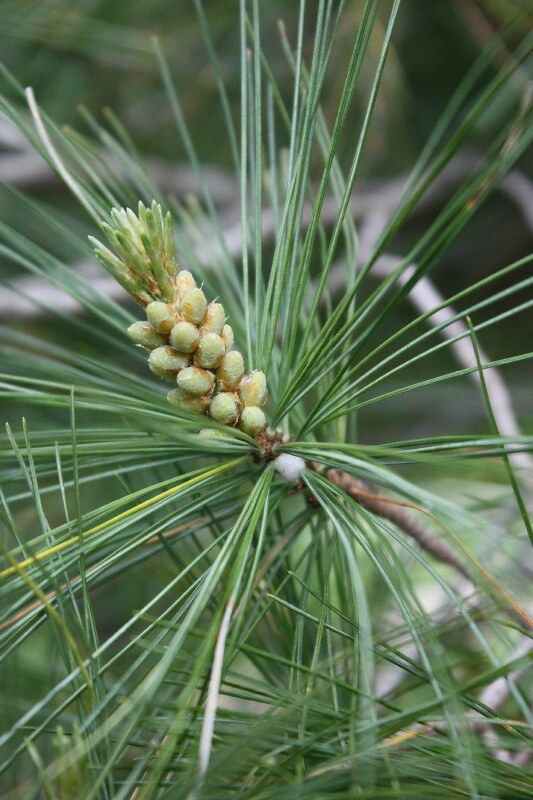The image showcases a close-up of a plant or tree branch that closely resembles an evergreen, such as a pine or cedar. The central branch extends from the lower right to the center, displaying a brownish stem adorned with numerous fuzzy, tan, and yellowish seed-like bulbs. These bulbs are clustered together and bear a striking resemblance to tiny pineapples. Surrounding the bulbs are dark green, spiky needles that extend in various directions, reminiscent of pine needles. Additionally, some light green, grass-like needles are visible near the bottom of the image. In the background, there are a few bare wooden branches without leaves, further emphasizing the primary branch's texture and color akin to a Christmas tree branch.